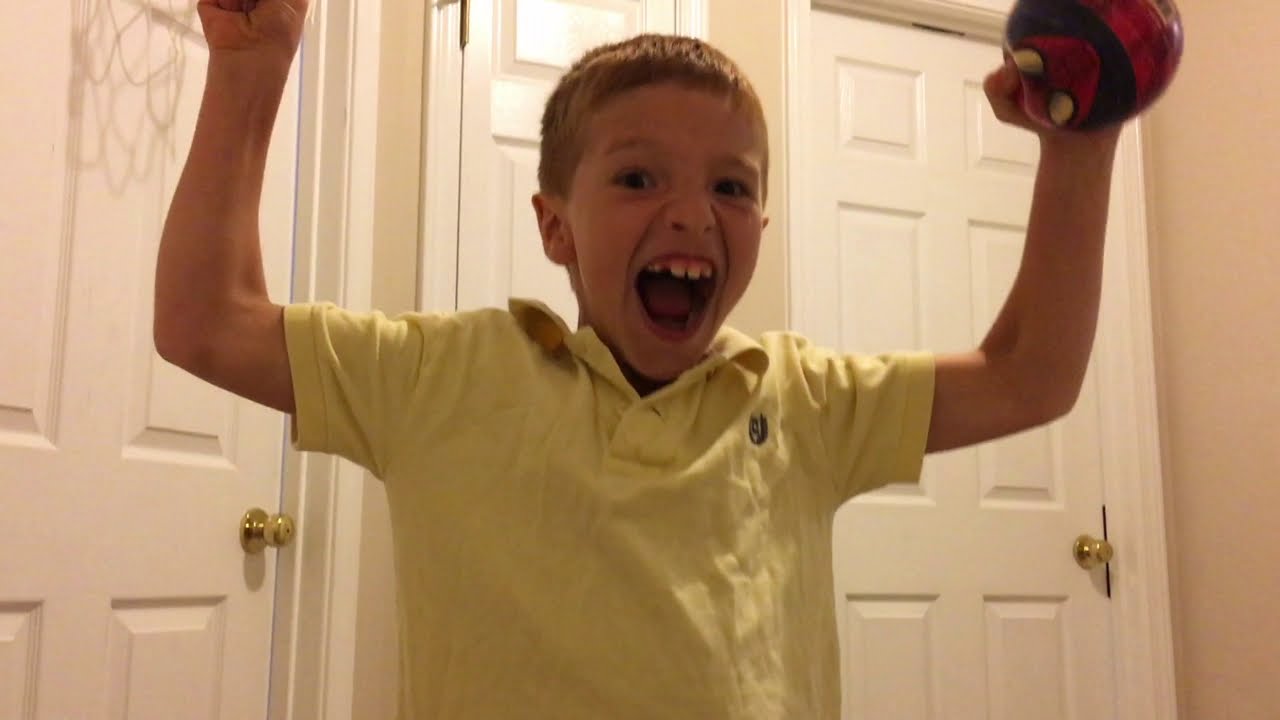In the image, a young boy, around six to eight years old, stands in the foreground, radiating excitement. He has short, blondish brown hair combed forward and is wearing a light yellow polo shirt with a small logo on the left breast. His arms are bent at shoulder level, his hands raised in the air, palms facing forward. In his right hand, he proudly holds a small Spider-Man basketball, red with white eyes and blue accents.

The boy's face is a picture of elation—his mouth gaping wide open as if he's yelling or cheering, with visible gaps where some of his teeth are growing in. This animated expression suggests he may have just made a basket in an exhilarating indoor game.

Behind the boy are three white doors, each adorned with gold doorknobs and latches. The door to the left also displays a discernible shadow or reflection of a basketball net, possibly indicating his recent successful shot. The surrounding walls are a tinted cream or tan color, adding to the warm, homey atmosphere of the scene.